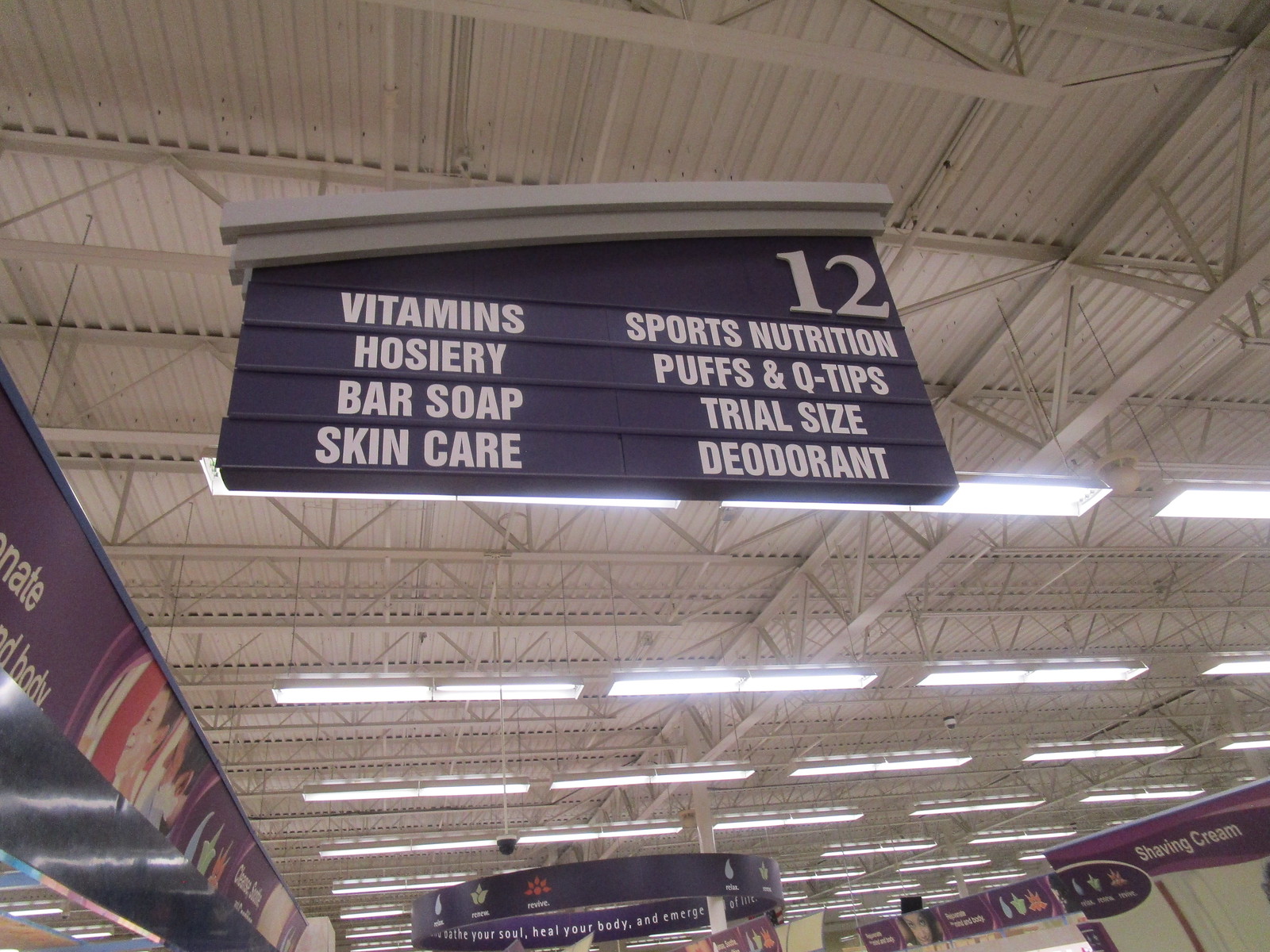The image depicts the interior ceiling of a commercial store, characterized by white panels accentuated with white structural bars and rectangular industrial lights suspended by black rods. Central to the image, a large aisle marker banner is visible, with a distinct gray top transitioning to a blue rectangle with white text. This banner categorizes the sections of Aisle 12, featuring "12" in the upper right corner. The left side of the banner lists items such as "Vitamins," "Hosiery," "Bar Soap," and "Skin Care," while the right side includes "Sports Nutrition," "Puffs and Q-tips," "Trial Size," and "Deodorant." Additionally, a purple banner with white lettering indicating "Shaving Cream" is visible in the bottom right corner of the image. The organized ceiling layout, with its suspended banners and lights, clearly marks the different sections, guiding shoppers efficiently through the store.